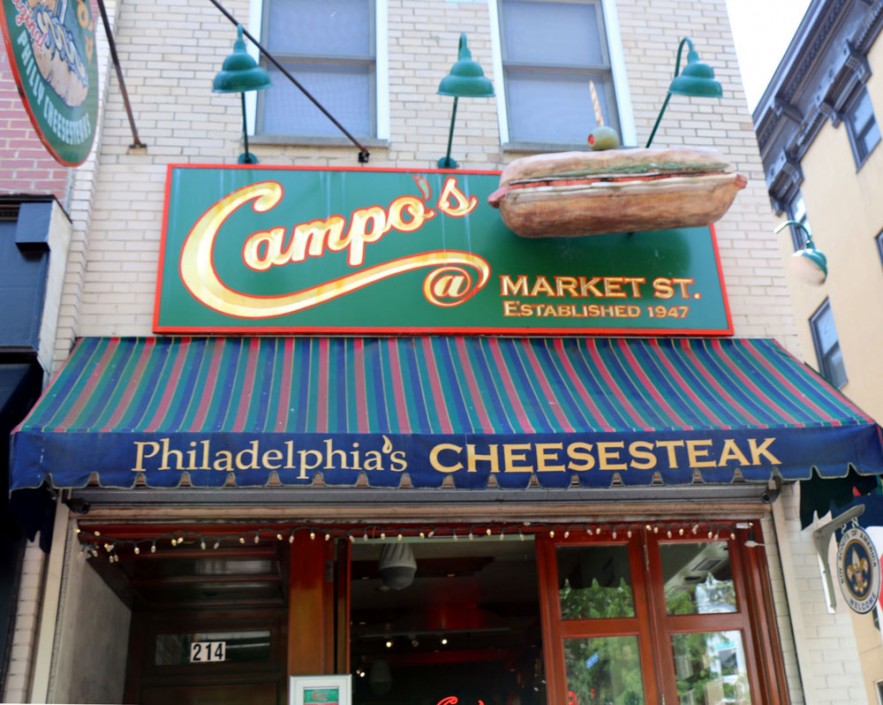The image captures the façade of a restaurant in a tall, tan-brick building. Prominently featured is a large sign at the top with an orange square border, a green background, and yellow cursive lettering reading "Campos at Market Street, established 1947." Above the text is a sculpture of a hot dog with an olive on a toothpick. Green lights hang down from long arms above this sign. Below the sign is an awning with staggered orange, green, and blue stripes, and "Philadelphia's Cheese Steak" written across the bottom in yellow text. The lower portion of the storefront includes brown doors with glass panels and the number "214" displayed in a white rectangle. The building frame appears wooden, with some window panels visible on the right side. The image is taken in landscape orientation, highlighting the detailed and vibrant exterior of the restaurant.